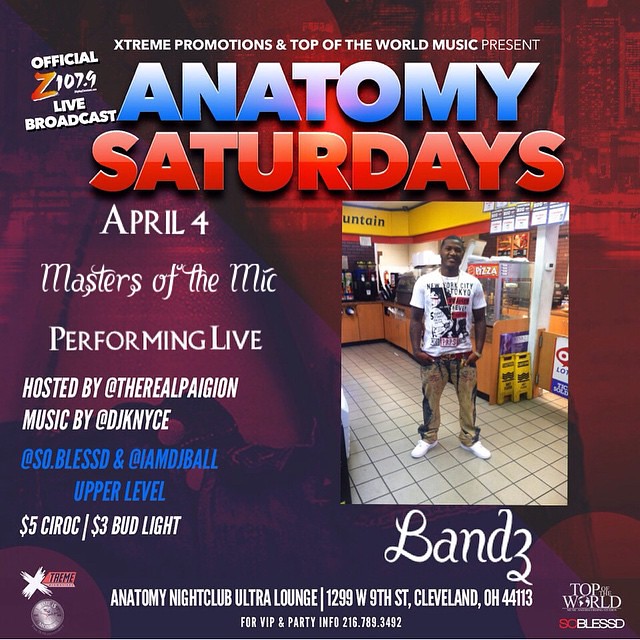Join us for "Anatomy Saturdays," brought to you by Z 107.9's live broadcast, Extreme Promotions, and Top-of-the-World Music, on April 4th. This event features the "Masters of the Mic" performing live, with hosting by @TheRealPA on Instagram. Enjoy music by @DJKNYCE, @So.Blessed (without the second 'e'), and @IAmDJBall. 

The event takes place at Anatomy Nightclub and Ultralounge, located at 1299 West 9th Street, Cleveland, Ohio, 44113. 

Experience great drink specials including $5 for Rock and $3 for Bud Light on the upper level.

For VIP services and party information, please contact 216-789-3492. Don’t miss out on this electrifying night!